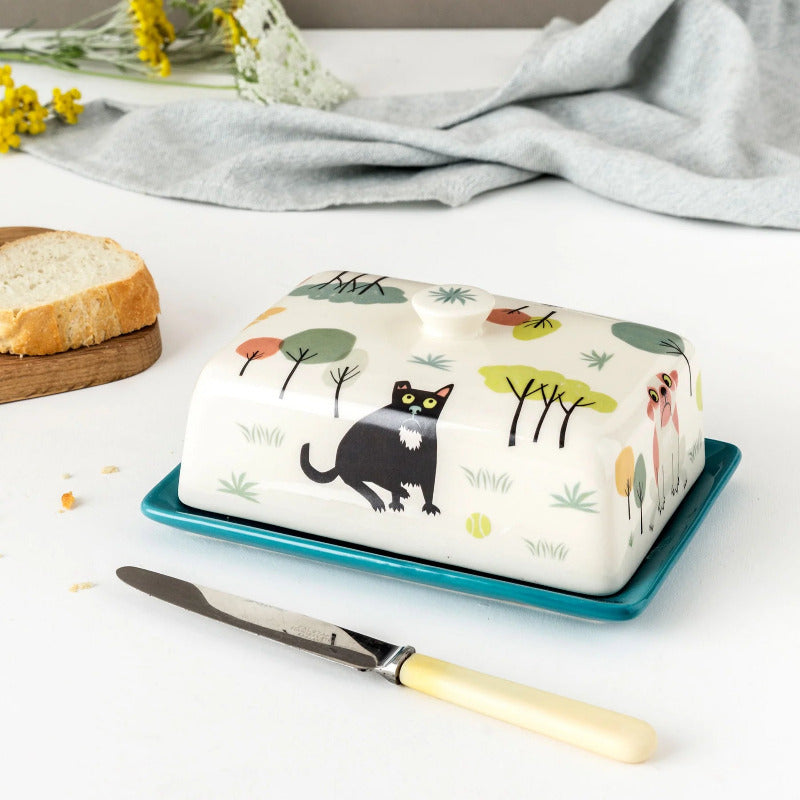In this indoor photograph, the focal point is a charming butter container situated centrally in the frame. The container features a ceramic, circular lid adorned with delicately painted designs, including abstract trees in hues of yellow, green, and blue, as well as whimsical depictions of a black dog, a white dog with pink ears and accents, and potentially a cat with green eyes. The base of the butter dish is a striking bluish-teal color. To the left, the scene extends onto a rustic brown wooden cutting board holding two slices of bread. A knife with an ivory or yellow handle rests in front of the butter container, its blade pointing left. The background comprises a folded, grayish-colored cloth and a beautiful bouquet of yellow flowers in the upper left corner, which adds a fresh, lively element to the neutral white tablecloth that covers the table.